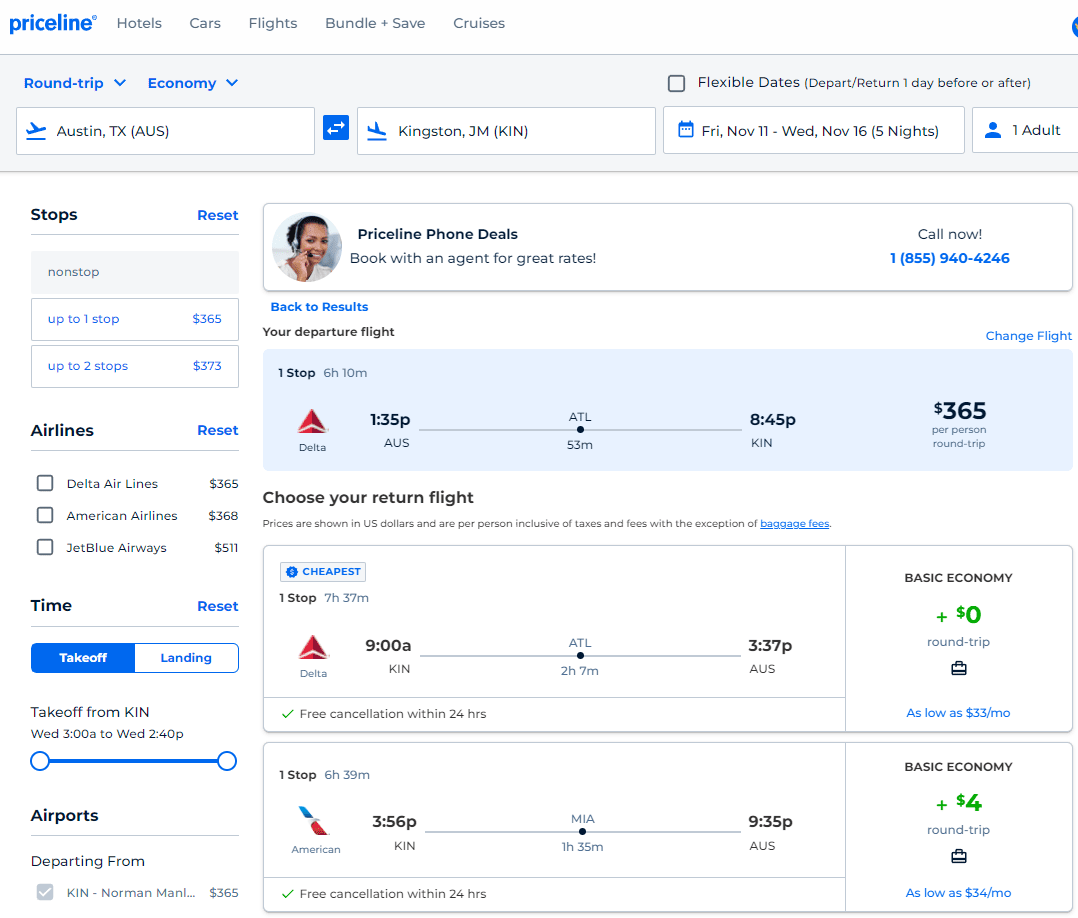Here is a cleaned-up and detailed caption for the image described:

"In this screenshot, Priceline displays airfare results for a round-trip economy flight from Austin, Texas to Kingston, Jamaica. The selected itinerary is for one adult, departing on Friday, November 11th, and returning on Wednesday, November 16th. The chosen departure flight is operated by Delta Airlines, with one stop, lasting 6 hours and 10 minutes, priced at $365. The return flight, also with Delta Airlines, includes one stop and has a duration of 7 hours and 37 minutes. The basic economy round-trip fare is noted as $365, with an option to finance for as low as $33 per month. Additionally, there is an alternative return flight option from American Airlines, featuring one stop and a duration of 6 hours and 39 minutes, priced slightly higher at an additional $4."